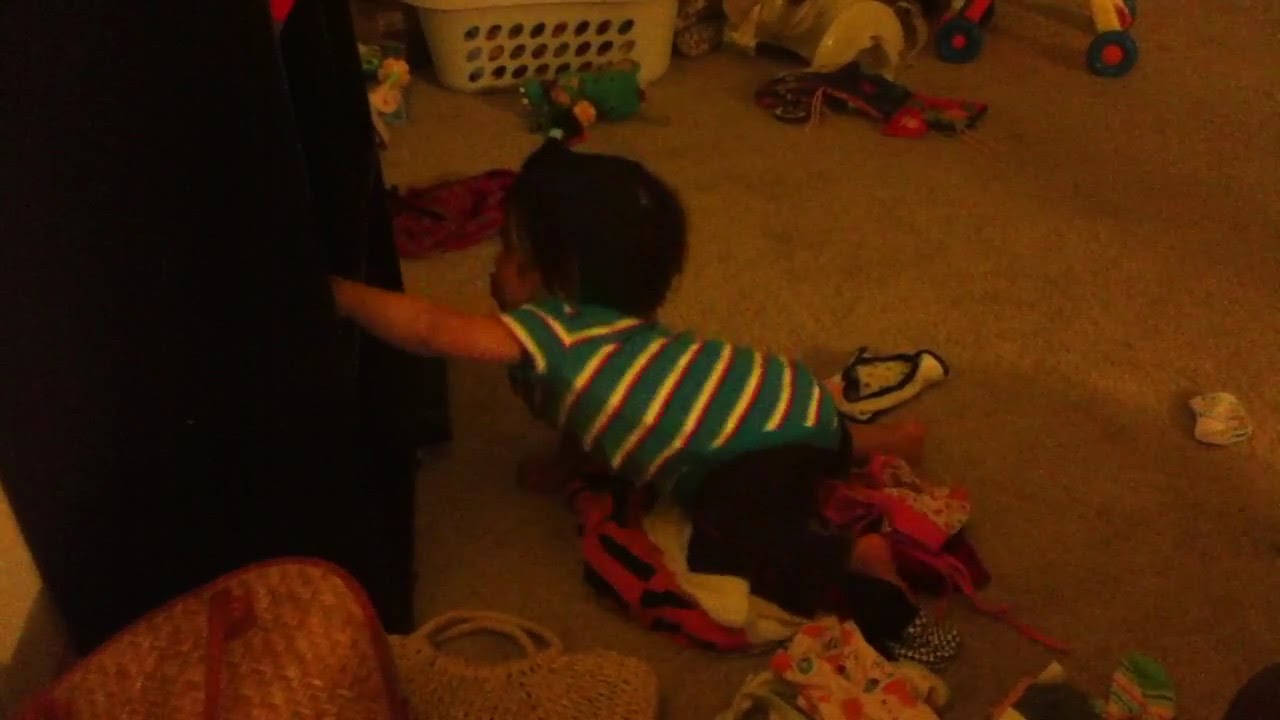In the warmly lit interior of a room, likely a bedroom or living room, a small child, approximately one to two years old, is prominently seen crawling on a beige carpet. The child has short black hair styled in a bob and is dressed in a green, white, and pink striped shirt, with black pants. The child's hand is reaching into an open dresser drawer on the left side of the image, surrounded by toys and clothes scattered across the floor. A small plastic basket, a basket purse, and various baby paraphernalia, including parts of a toy horse with wheels, are noticeably spread out around her. Additional items such as a laundry basket can be seen in the background, indicating a space filled with playful, everyday chaos. The room appears to be dimly lit, with the primary source of light coming from a lamp visible in the scene, suggesting it is nighttime.